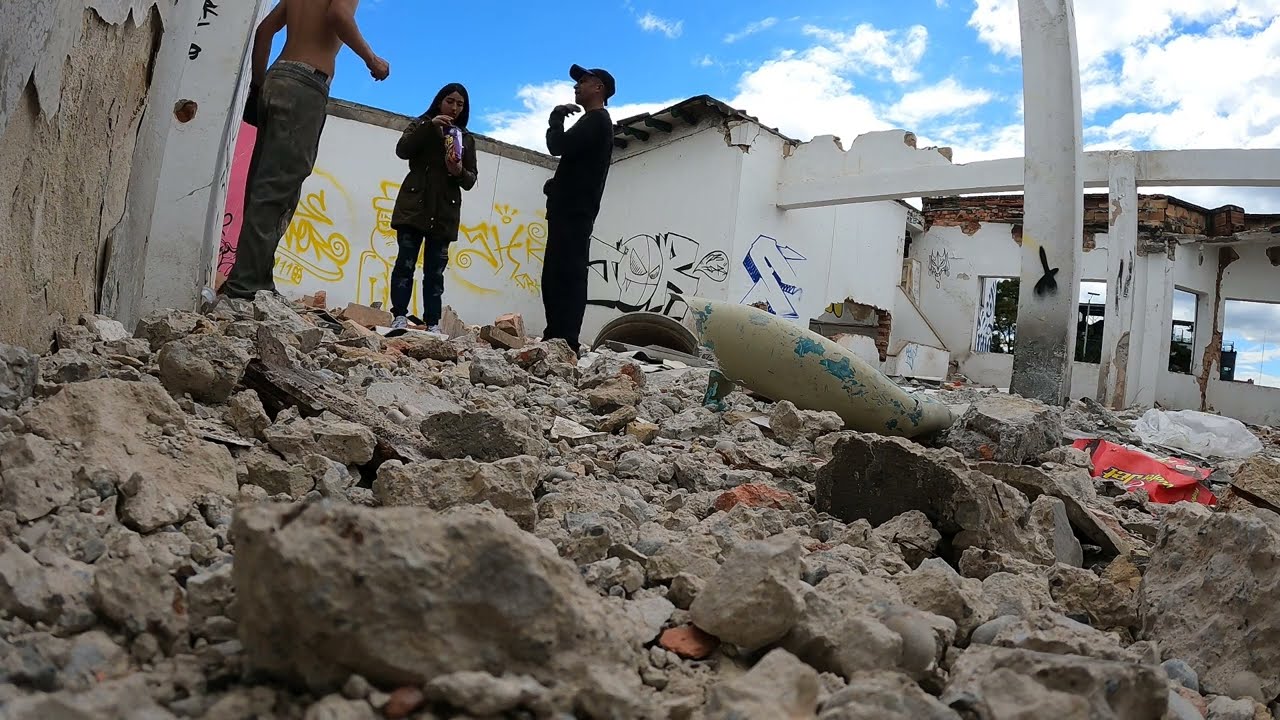In this detailed image, taken from ground level, we see a scene of complete destruction and disrepair. The foreground is dominated by a chaotic mix of rubble, consisting of shattered concrete and rocks from a once-standing structure. The photo, captured outdoors during the day, reveals a sky dotted with fluffy clouds above the ruins. Amidst the debris, a partially standing white building is visible, bearing colorful graffiti in shades of yellow, black, and blue, and a few broken columns and beams.

On top of the rubble, three individuals can be seen. To the left stands a shirtless man clad only in long pants. At the center is a woman in a black jacket and pants, casually eating potato chips from a bag. To her right stands another man dressed in dark clothes and a baseball cap, engaging in conversation or gestures. The scene starkly depicts a moment frozen in the aftermath of destruction, with the desolated structure and its remnants set against an open, cloud-filled sky.